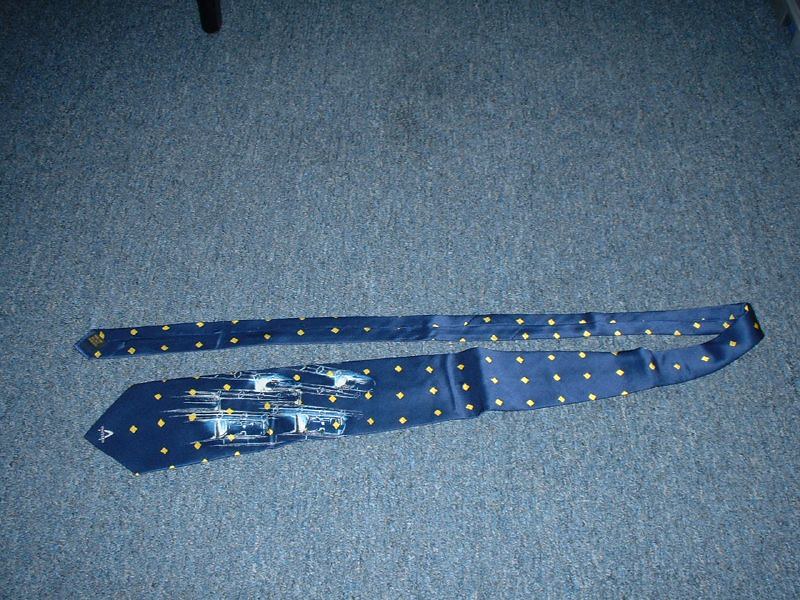This photograph captures a detailed scene of a navy necktie with small, yellow diamond-shaped patterns, laying on a grayish carpet, seemingly in a dimly lit hotel room illuminated by flash photography. The tie is open and stretched out on the floor, revealing a white smudge or stain prominently across its front. The gray carpet, appearing synthetic and inexpensive, serves as the backdrop, with a distinct black table leg visible in the top left corner of the image. The tie's yellow diamond patterns are arranged in rows, starting with three diamonds per row which then transitions to a single diamond per row further down. Additionally, there is an 'A' shaped logo in white near the bottom of the tie, situated above the noticeable white stain.